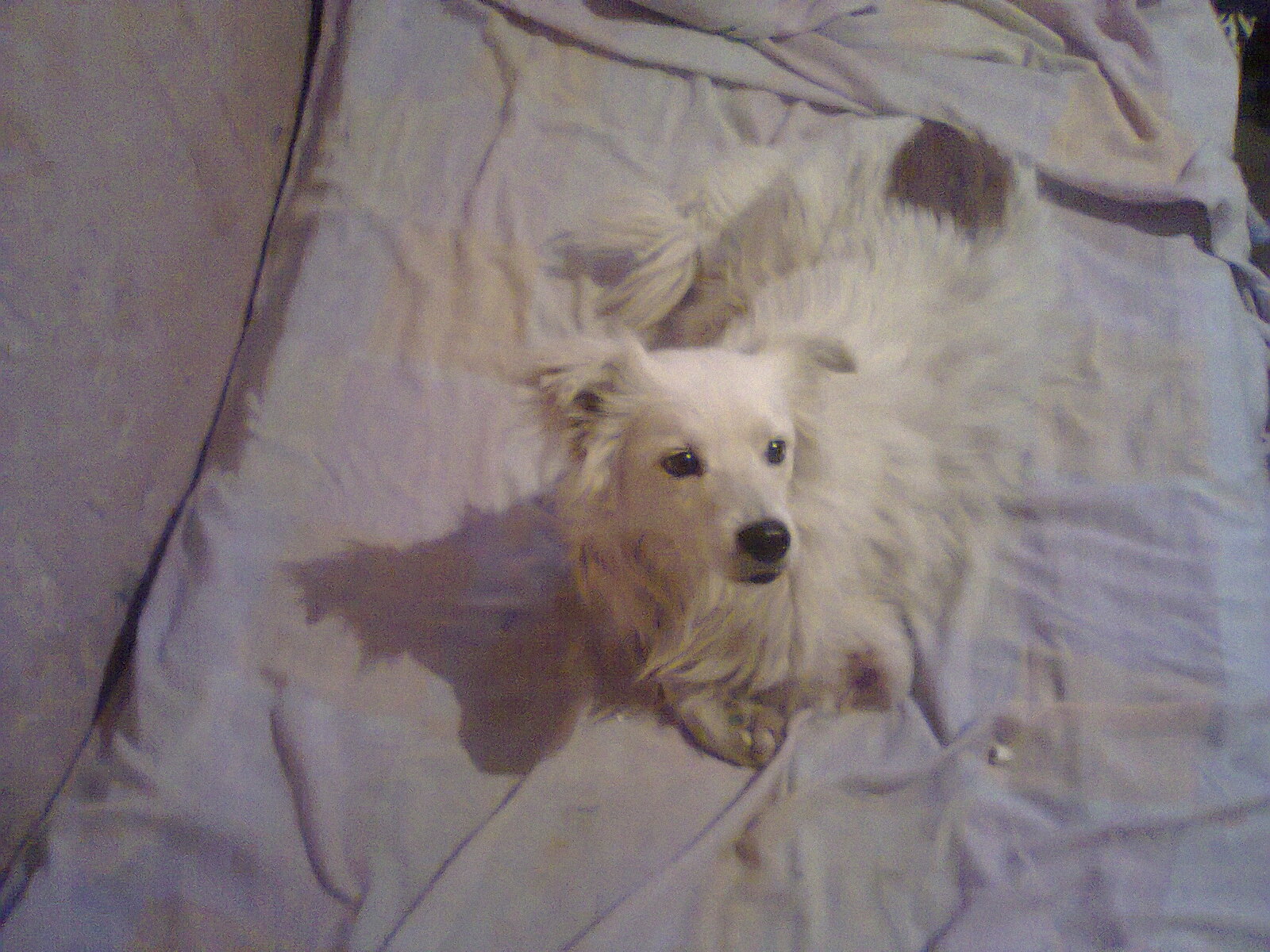This image is a wide rectangular photograph taken indoors, roughly six inches wide and four inches tall, with a slightly grainy and blurry quality. The central focus is a small, fluffy dog with predominantly white, long fur that transitions to darker shades, particularly on its hindquarters, where there is a distinct rectangular patch of black. The dog has floppy, white ears and dark eyes, which are looking towards the right. Its nose is black, and its fur around the face is shorter compared to the fluffier, more pronounced fur on the ears, chin, and the sides of its face. The dog is laying down on a checked blanket—light purple with light yellow squares—covering what might be a gray couch. The blanket appears wrinkled and bunched up in the top right and bottom right corners, while a light purple cushion is visible in the top left corner. The dog's front paws are curled underneath its body, and a shadow of its head can be seen on the bottom left side of the blanket.